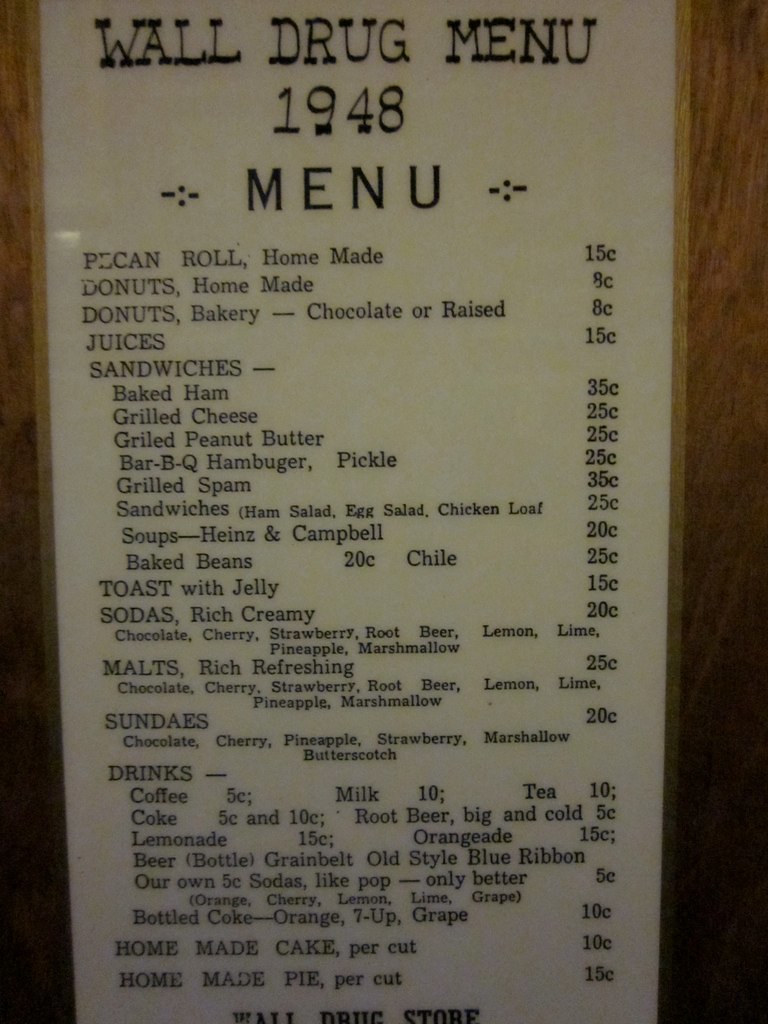This image features a vintage restaurant menu from Wall Drug, dated 1948, displayed on a wooden table. The menu highlights a variety of pastries, breakfast items, beverages, and sandwiches. Offerings include pecan rolls, donuts, and an assortment of juices. A diverse sandwich selection is available, featuring options like baked ham, grilled cheese, grilled peanut butter, barbecue, hamburger with pickle, grilled Spam, ham salad, egg salad, and chicken sandwiches. Soups from Heinz and Campbell's, as well as baked beans, are also listed. Toasted jelly sandwiches and a rich assortment of sodas, available in flavors such as chocolate, cherry, strawberry, root beer, lemon-lime, pineapple, and marshmallow, are prominently featured. Additionally, the menu includes malts and sundaes, as well as drinks like coffee, various Coca-Cola products, root beer, and orangeade. There is also a selection of beers including Greenbelt, Old Style, and Blue Ribbon. To complement the meal, homemade cake and pie are offered, completing the nostalgic culinary journey.